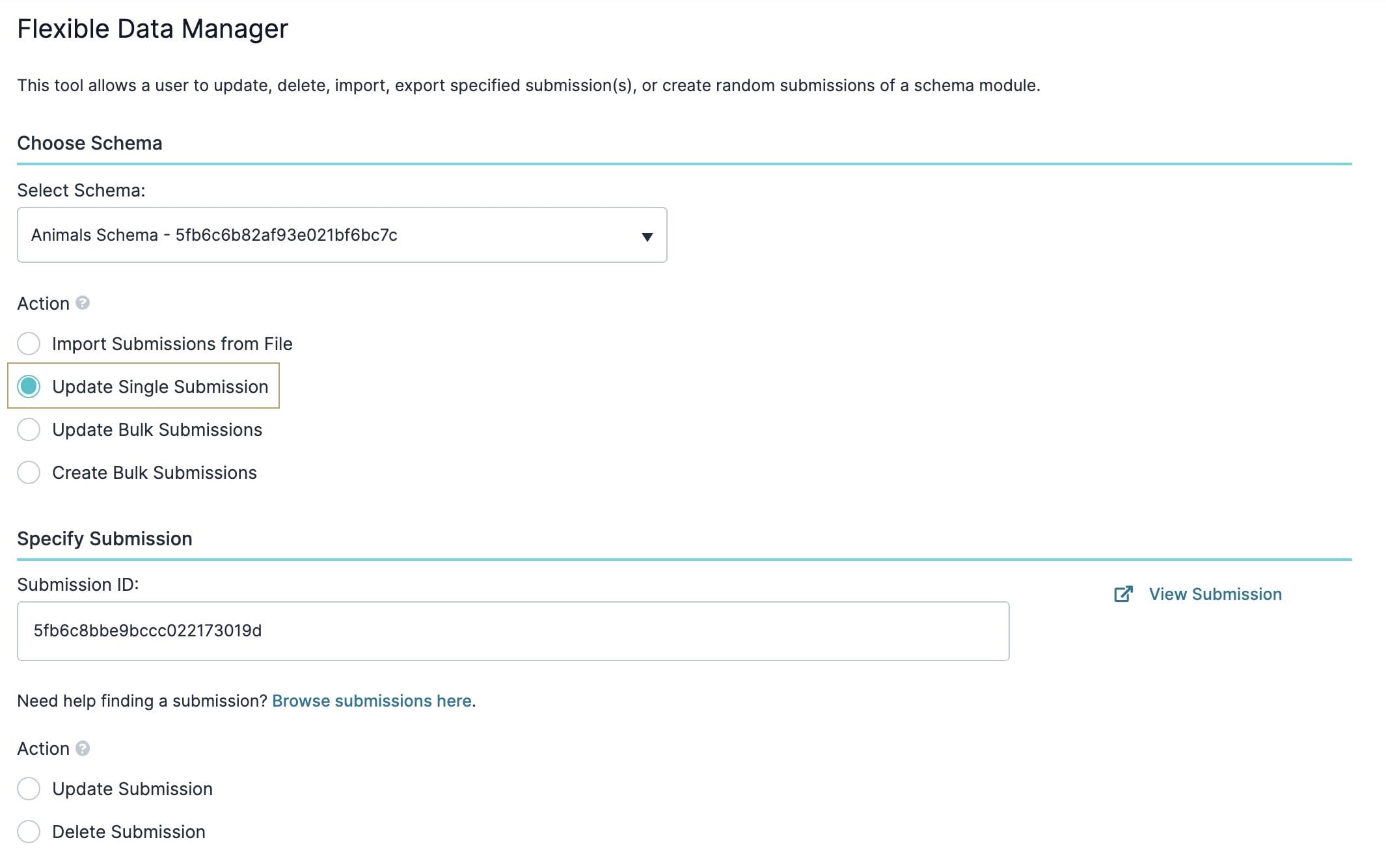The image shows a website interface centered to the left side of the screen. At the top, a bold black header reads, "Flexible Data Manager." Below this, in thinner black text, it states, "This tool allows a user to update, delete, import, export specified submissions, or create random submissions of a schema module."

Another bold black header below reads, "Choose Schema," separated by a long blue line from the subsequent section. Underneath, it says, "Select Schema" with a drop-down menu box where the "animal" schema is selected, accompanied by an alphanumeric code. 

Next, there is a section titled, "Action," offering four options: "Import Submissions from File," "Update Single Submissions," "Update Bulk Submissions," and "Create Bulk Submissions." The "Update Single Submissions" option is selected, indicated by a highlighted box and a blue dot.

Further down, a bold black header reads, "Specify Submission," followed by another blue separating line. This section includes a box for the "Submission ID" with an alphanumeric value entered. On the right side, there is a hyperlink labeled "View Submission."

Under this box, in black text, it reads, "Need Help Finding a Submission?" with a hyperlink that says, "Browse Submissions Here." At the bottom, it says "Action" with two available options: "Update Submission" or "Delete Submission."